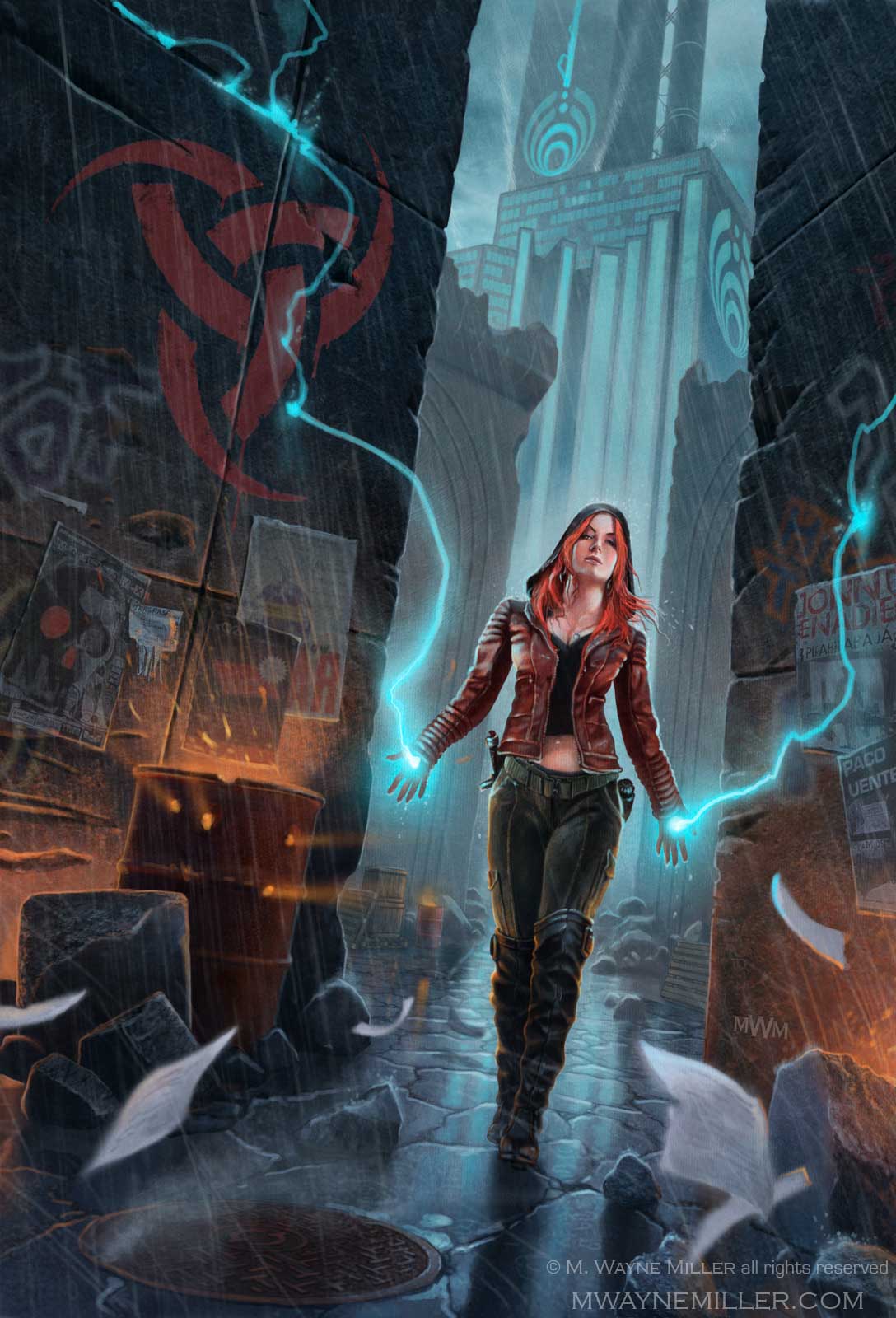The poster for the movie features a striking image of a young redheaded woman exuding an aura of power and resilience. She is walking towards the viewer, clad in a maroon leather jacket, a black midriff-baring top, and dark pants paired with over-the-knee boots. Adorning her outfit is a knife sheathed at her right hip. Her hair flows as she strides confidently on a wet gray cobblestone path, littered with debris and broken pieces of the surroundings, including a visible sewer grate toward the bottom left.

The setting is amidst two gray brick buildings, where electric blue arcs of lightning emanate from her hands, crawling up the walls, illuminating the gloomy, rain-soaked scene. A fire burns in a nearby 50-gallon barrel on her right side, casting an eerie glow. In the background, a tall building looms through the rain, adding to the sense of dystopian tension. The artist’s name, M. Wayne Miller, and his website, mwaynemiller.com, are inscribed at the bottom right, indicating the piece's craftsmanship. The image is vibrant, almost abstract, with a vivid and chaotic background bathed in blue light, suggesting a fantastical or video game-like quality to the scene.